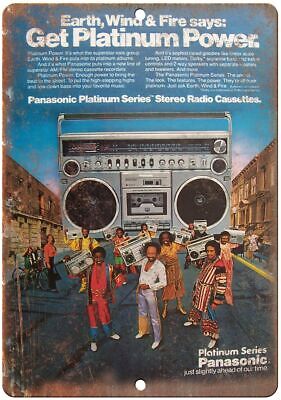This image is a vintage advertisement placard for Panasonic boomboxes featuring the band Earth, Wind, and Fire. At the very top, written in white letters against a backdrop of a blue sky with clouds, it says, "Earth, Wind, and Fire says get Platinum Power." There is some small, indistinct text beneath this line, followed by the prominent text, "Panasonic Platinum Series Stereo Radio Cassettes." The focal point of the advertisement is a large, silver boombox stereo, complete with a black dial, two large black speakers, two smaller black speakers, a central cassette holder, and numerous buttons and switches. In front of the boombox stand several smiling African-American individuals dressed in colorful outfits: one in bright orange, one in blue pants with a white shirt, and another in a striped outfit. Each is holding a Panasonic boombox slung over their shoulder. They are positioned in the middle of a street flanked by brown buildings on either side. At the bottom right of the placard, it states, "Platinum Series Panasonic—just slightly ahead of our time," with some weathering and rust visible around the edges of the sign.